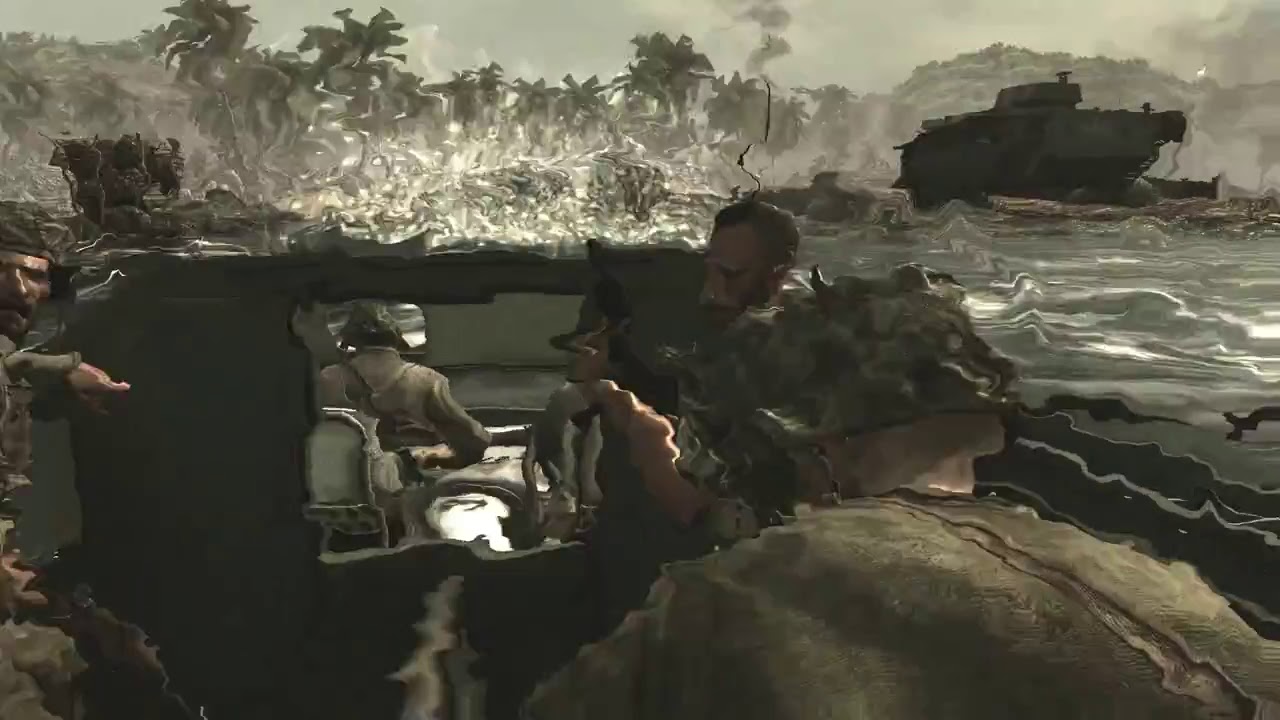In this heavily distorted and wavy screenshot from a video game, we are given an immersive view from inside a military vehicle. The vehicle is crowded with several soldiers dressed in green camouflage fatigues, some wearing helmets and others holding high-caliber weapons. The scene has a green color theme and appears to take place in an outdoor, tropical environment. In the distance, we can spot a tank and an array of palm trees against a hill covered with lush greenery. The sky overhead is notably dark, adding a foreboding atmosphere to the scene. The entire image has been warped with a strange, mushroom-trip-like filter, giving it a surreal, almost psychedelic effect. The rectangular frame of the screenshot suggests that the vehicle might be on water, contributing to the chaotic and blurry nature of the visual. Despite the poor quality and the distortion, the scene captures a tense military moment amid the vivid backdrop of a tropical battlefield.